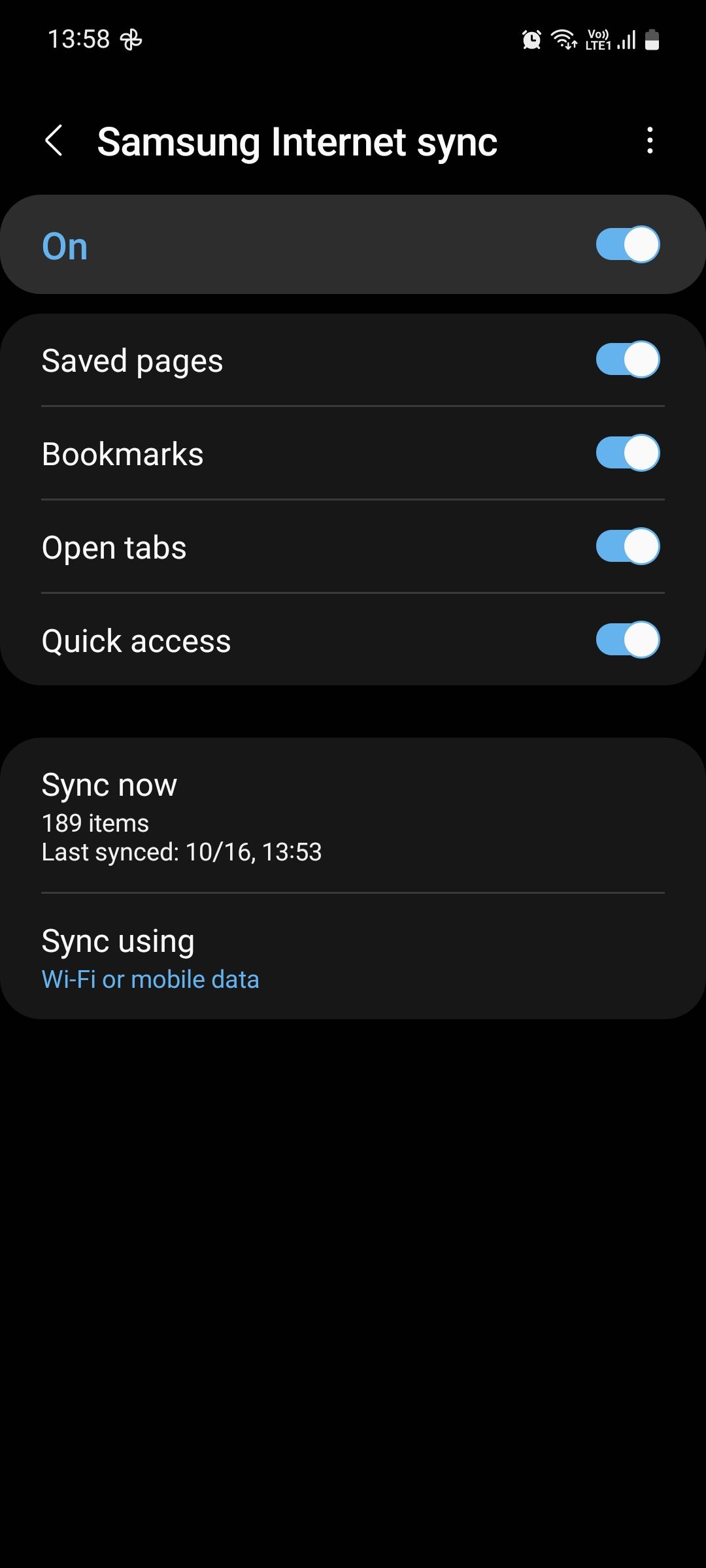The image is a screenshot set against a solid black background depicting settings within a Samsung Internet browser. In the upper left corner, the time is displayed as 13:58. The upper right corner shows the Wi-Fi is connected, LTE 1 is active with full bars, and the battery is at half capacity.

The main section presents the Samsung Internet Sync settings in white text. Below that, in blue text, it indicates "On" with the toggle switch turned on. Subsequent options include:

- Saved Pages: Toggle on
- Bookmarks: Toggle on
- Open Tabs: Toggle on
- Quick Access: Toggle on

Below these options is a "Sync Now" button with an accompanying smaller white text indicating "189 items. Last synced: 10-16-13-53." A light gray stripe divides this section from the footer, which states "Sync using Wi-Fi or mobile data" in white text.